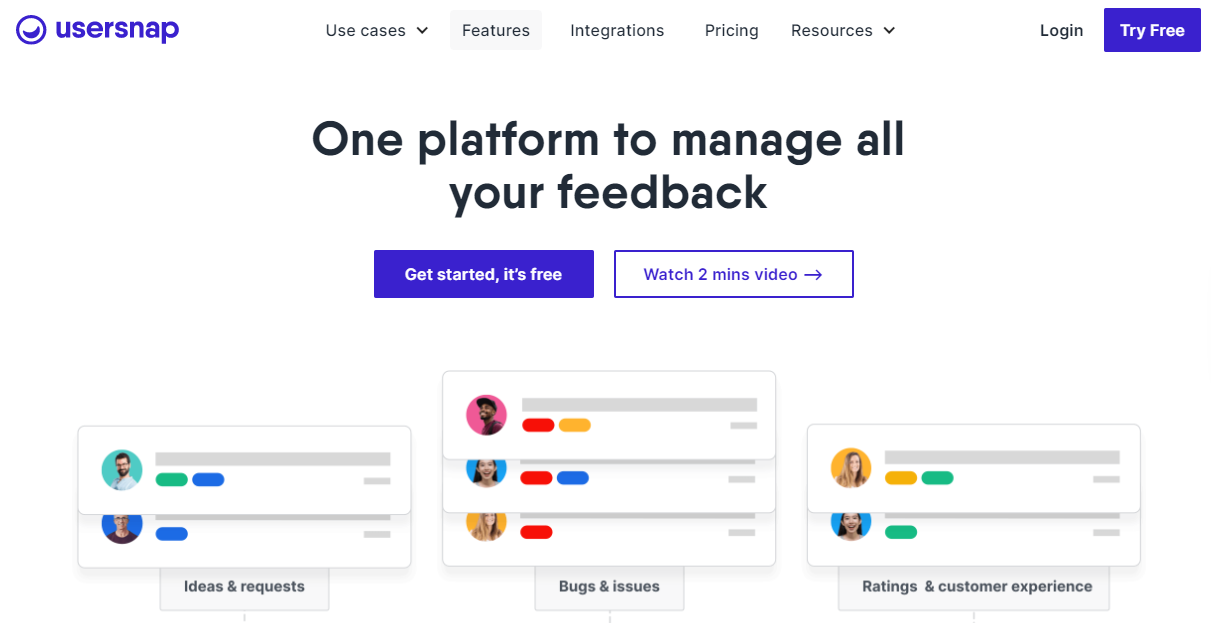A screenshot from the UserSnap website prominently features their logo in the upper left corner—a circular emblem with a minimalist smile, but no eyes, rendered alongside the company name in a purplish-blue hue. The site’s navigation bar at the top lists key sections: "Use Cases," "Features," "Integrations," "Pricing," "Resources," and a "Login" option. A conspicuous "Try Free" button, set in a bluish-purple box, invites visitors to engage with the platform.

Just below, the main headline boldly states, "One platform to manage all your feedback," in black font. Accompanying this headline is a call-to-action button that reads "Get started, it's free," situated within a purplish-blue box. Adjacent to this is an option to "Watch two-minute video," marked by a right-arrow icon.

Further down the page, three distinct sections showcase blurred content, representing user-generated posts categorized into different types of feedback. The left section, labeled "Ideas and Requests," displays two posts. The middle, titled "Bugs and Issues," contains three posts, while the right section, "Ratings and Customer Experience," holds a varying number of posts.